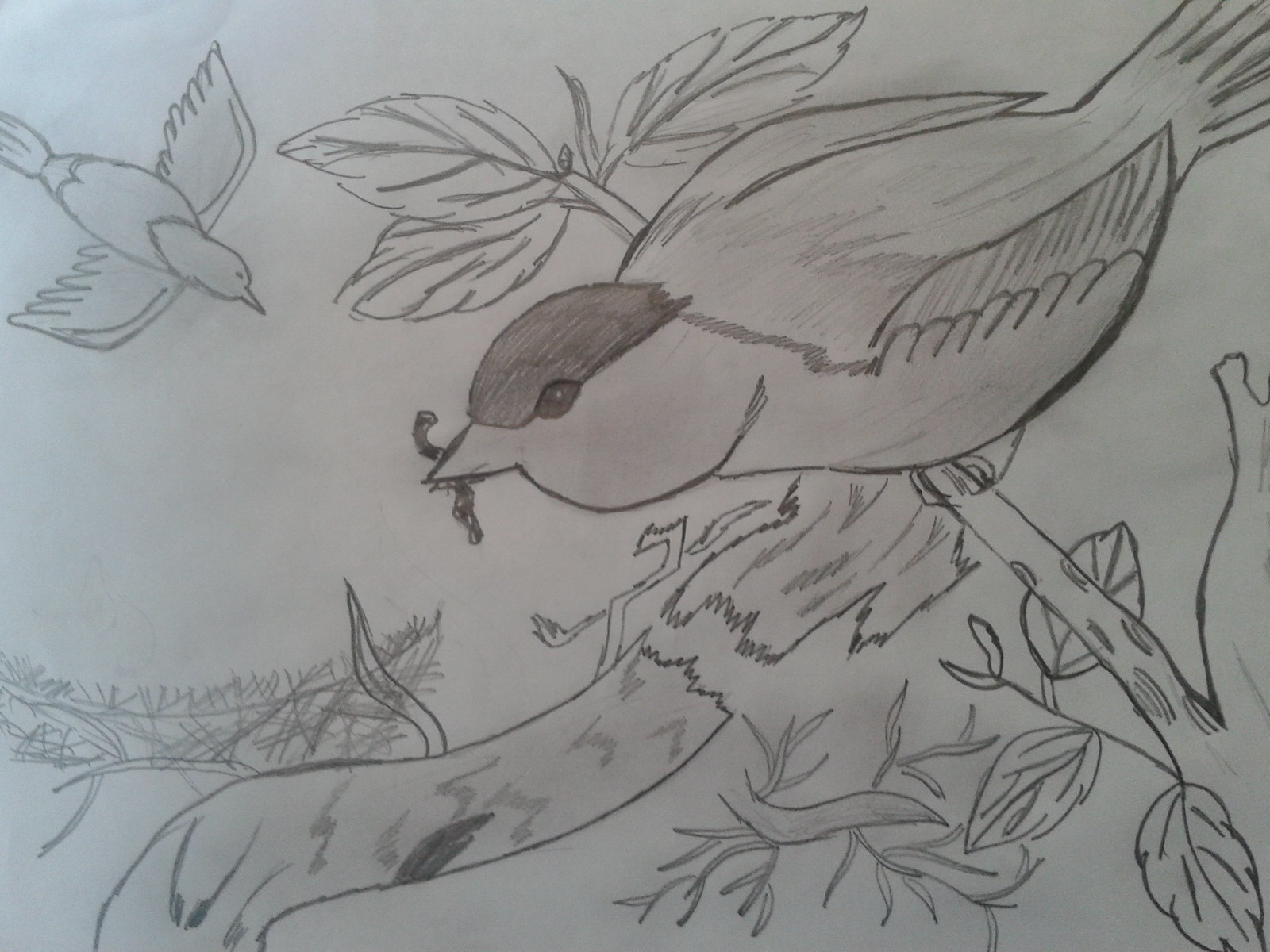This detailed pencil drawing features a central bird, resembling a chickadee or sparrow, perched on a tree branch. The bird, rendered in shades of black, white, and gray, has distinct dark markings on its head and stripes on its wings. It is holding a worm in its beak, facing downwards to the left, with its tail extending towards the top right corner of the image, slightly off the page. The branch it rests on has several leaves, comprising two pointing downwards and one upwards. 

In the background, extending towards the upper left corner, the broken tree trunk continues, accompanied by additional leaves and smaller limbs jutting out. Another bird appears in the upper left, drawn with simple outlines and minimal details, such as marked eyes and a slight breast marking. This secondary bird is depicted as flying, with wings spread wide and the underside visible, giving the impression of it soaring below the main bird. 

Below the primary bird, the tree branch appears broken with fragments and bark scattered beneath, adding to the sense of a natural setting. The detailed texturing and meticulous shading bring a lifelike quality to this serene woodland scene.